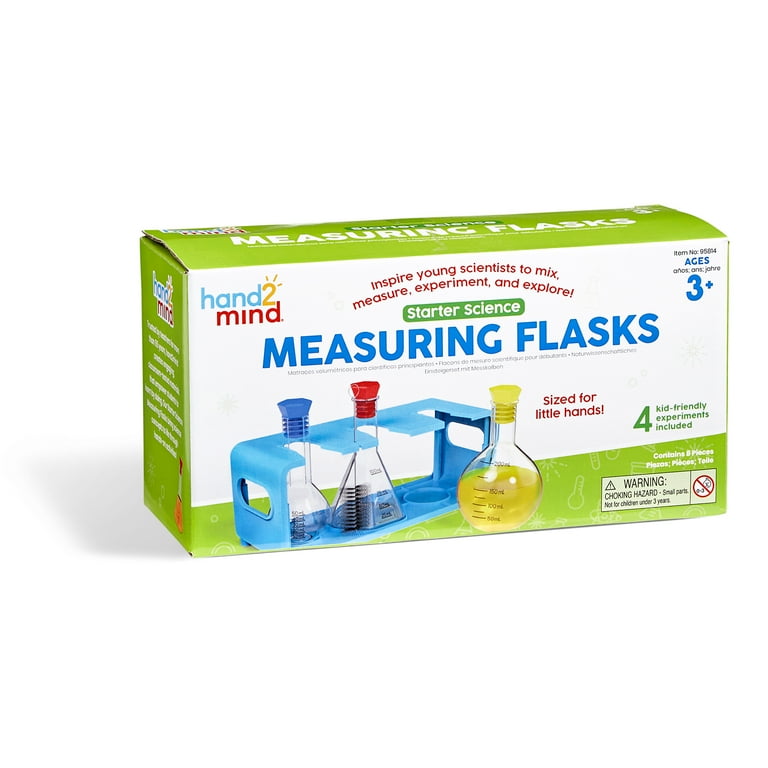This image showcases a rectangular cardboard box designed as a little science starter kit for kids, predominantly white at the front with green accents on the top and sides. The top portion features the text "Inspire young scientists to mix, measure, experiment, and explore" in red letters arranged in a hemisphere shape. Below this, in green letters against a white background, it reads, "Starter Science," and further down, "Measuring Flasks" is displayed in blue. The box displays an image of a blue plastic container holding three distinct flasks – one with a yellow topper, another with a red stopper, and the third with a blue stopper. It is specified that the set is "sized for little hands" and includes "four kid-friendly experiments". The right-hand side of the box shows a green number 4, indicating the number of pieces, and notes that the kit is suitable for ages 3 and up, with a warning about small parts posing a choking hazard for children under three years old. The front left of the box also features the brand name "hand2mind" and the text "ages 3+" prominently displayed.